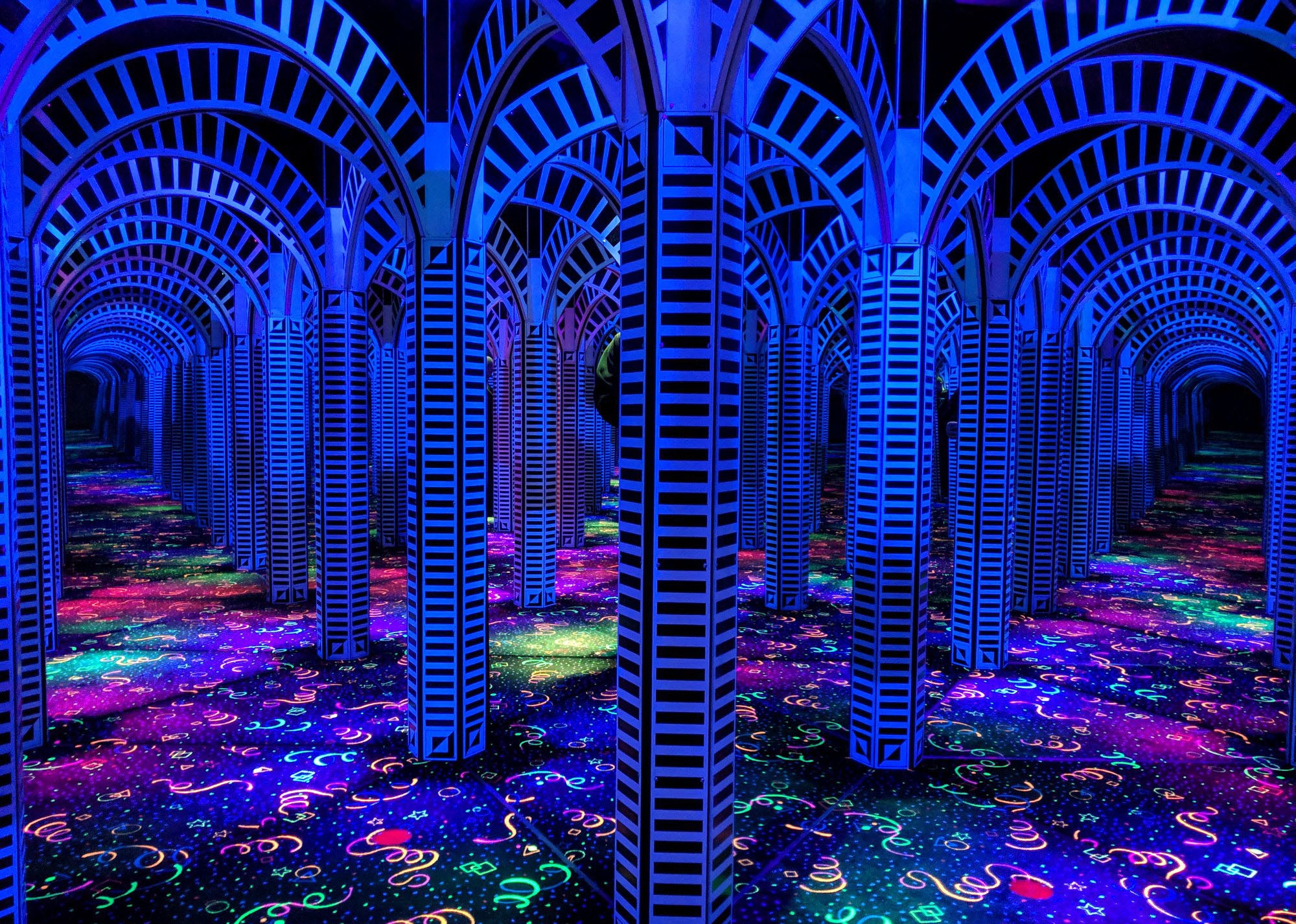The image appears to depict a vibrant and disorienting House of Mirrors, reminiscent of those found at carnivals and recreational attractions. The environment is predominantly dark, illuminated by neon colors that create a striking visual contrast. Two tunnels split off diagonally from the center, leading into dark hallways lined with large bluish-black striped archways and columns. The space is bathed in black light, accentuating the neon hues and creating an otherworldly glow. The floor is carpeted with swirling, colorful patterns—featuring greens, pinks, reds, yellows, blues, and purples—which add to the room's whimsical feel. At the center of the room, mirrors reflect these intricate designs and repeating archways, increasing the sense of depth and making navigation appear tricky. The overall setting is a maze of reflections, brightly colored shapes, and glowing structures that evoke the nostalgic allure and playful confusion of a classic fun house.